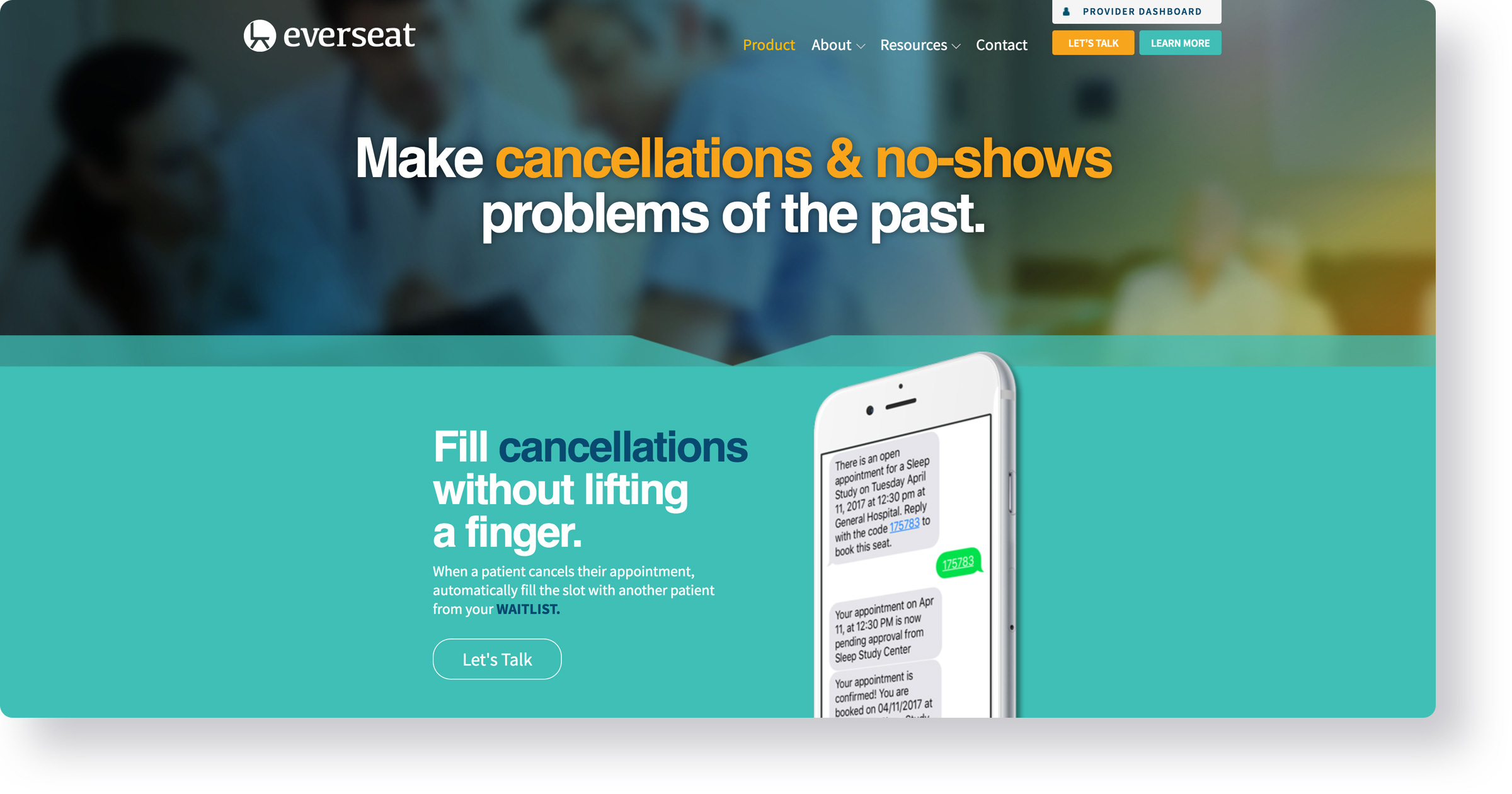Screenshot of Everseat Website (Promotional Image)

The screenshot features a promotional banner for the Everseat website. In the upper left-hand corner is a white circle containing a black icon resembling a desk chair and the brand name "Everseat" written in white, capitalized letters. To the right, the navigation bar includes links to "Product," "About," "Resources," and "Contact," alongside a "Provider Dashboard" button. There are two prominent call-to-action buttons: an orange "Let's Talk" button and a green "Learn More" button.

The main headline reads, "Make cancellations and no-shows problems of the past," displayed in white and orange text. Below it, a subheading states, "Fill cancellations without lifting a finger," explaining that when a patient cancels their appointment, Everseat automatically fills the slot with another patient from the waitlist. This message is reinforced with another "Let's Talk" button.

To illustrate the concept, there's an image of a white smartphone with a messaging interface on its screen. The screen shows a conversation with replies, giving a visual demonstration of the service in action. The background of the promotional area is a soothing teal or aqua color. At the top of the banner, there is an image of a healthcare professional wearing a stethoscope, engaging in conversation with several individuals in a room, adding a human touch to the digital service being promoted.